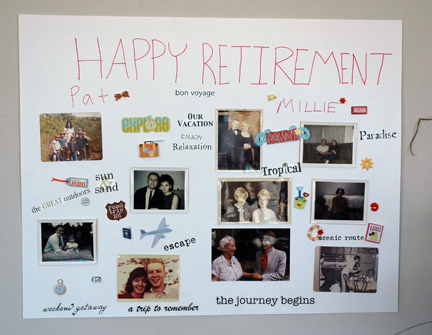This is a detailed photograph of a vibrant retirement poster titled "Happy Retirement Pat and Millie," prominently displayed in cheerful pink crayon-like writing. The poster is a heartfelt collage likely created for a retirement go-away party, celebrating the adventures and memories of Pat and Millie. It features around nine or ten nostalgic photographs, including a small picture of someone hiking, a couple dressed in formal attire embracing, and various images of couples enjoying different moments together. The collage also captures a picture of a woman from the 1950s, a family vacation, grandparents and a child in a kitchen, and someone relaxing on a couch. Scattered among the images are uplifting slogans like "Paradise," "Tropical," "Escape," "The Journey Begins," "A Trip to Remember," "Sun and Sand," adding a layer of warmth and excitement about the retirees' future adventures. The poster is further embellished with small pictures and trinkets, making it a cherished keepsake that encapsulates a lifetime of memories and anticipations for new beginnings.